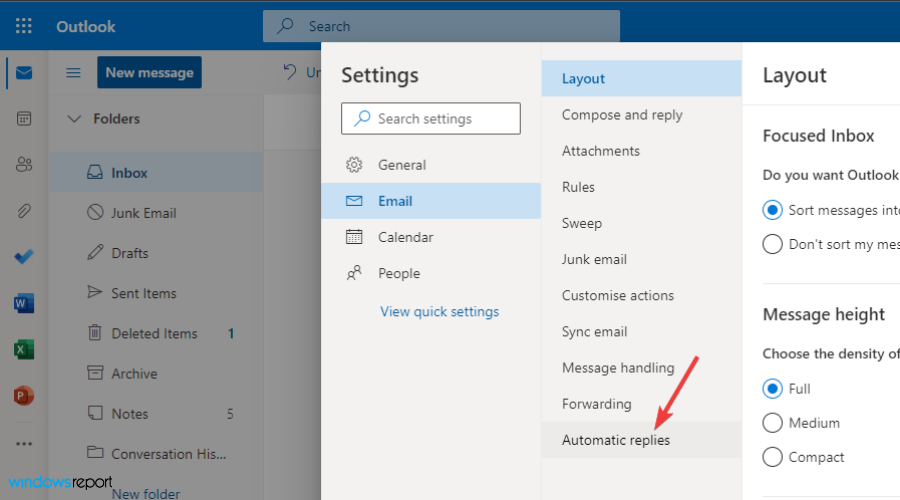The image depicts a screenshot of the Outlook email interface on a white background. The top of the interface features a blue header that contains a search bar and a hamburger icon. Adjacent to these elements is a blue rectangle with the text "New Message" prominently displayed in white.

On the left side of the screen, there is a list of folders including "Inbox" (which is shaded blue), "Junk E-mail," "Drafts," "Sent Items," "Deleted Items" (which has a notification indicator with the number one), "Archive," "Notes" (which has the number five next to it), "Every Conversation," and "History." There is also a "New Folder" option in blue.

Within the settings section, there is another search bar and categories listed as "General," "E-mail" (highlighted in blue), "Calendar," "People," and "Very Quick Settings" (in blue). Under this, options include "Layout" (highlighted in blue), "Compose and Reply," "Attachments," "Rules," "Sweep," "Junk E-mail," "Customize Action," "Sync E-mail," "Message Handling," "Forwarding," and "Automatic Replies" (highlighted in gray). A red arrow points to the "New Message" rectangle.

At the bottom, there is a layout section that includes "Focus Inbox" with text inquiring "Do you want Outlook?" There are two circles beneath this text. The first circle is shaded blue and appears partially cut off with the text "sort messages" starting with "INT." The second circle, which has "Don't sort my messages," also appears partially cut off with "MES" visible.